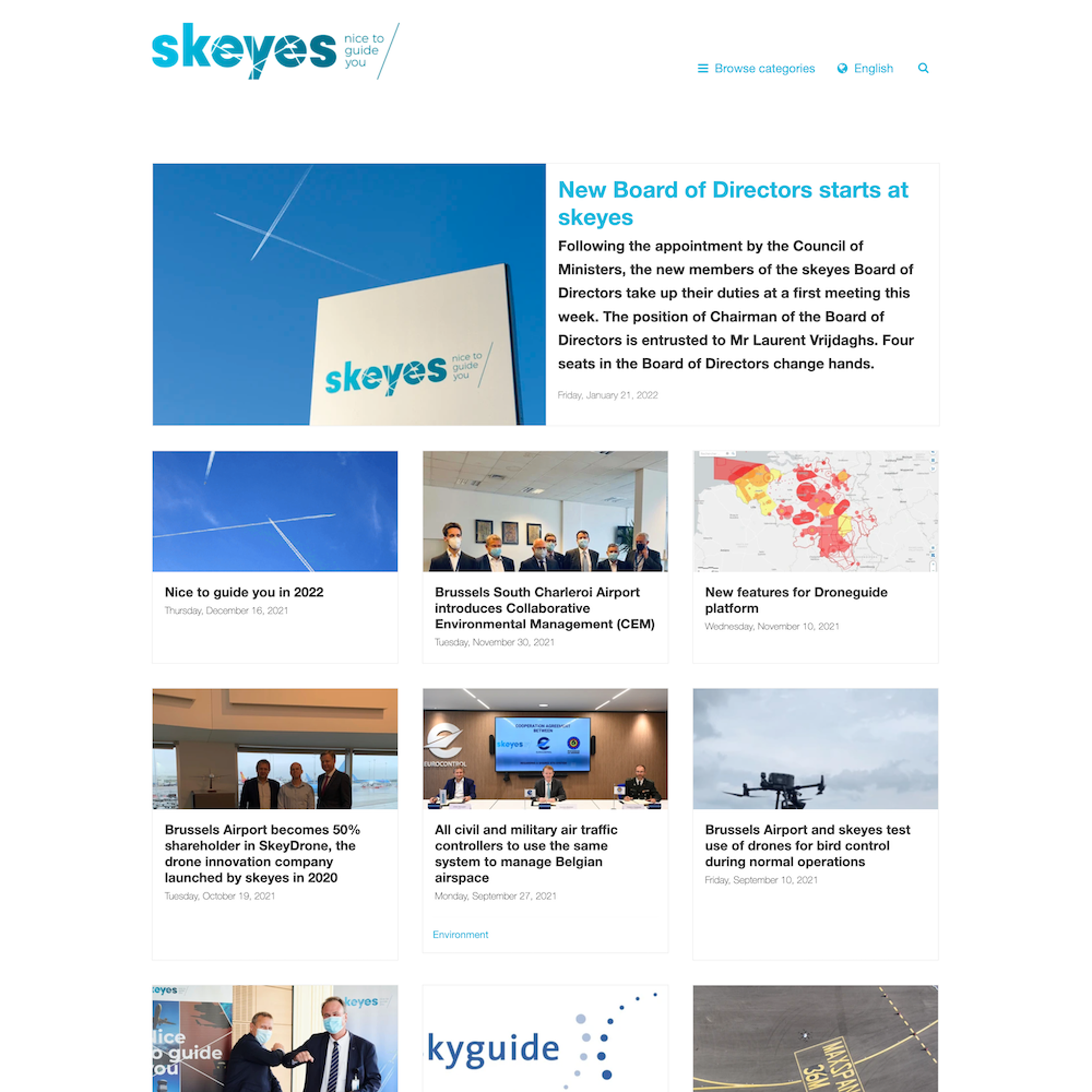**Caption:**

A screenshot from the Skyes (S-K-E-Y-E-S) application showcasing its user interface. The Skyes logo is displayed prominently in bold font against a gradient blue background that transitions from light blue on the left to medium blue on the right, adorned with white lines. On the right-hand side, there are options to 'Browse Categories,' 'English,' and a search icon.

The main section features various news articles. The top article headline reads: "New Board of Directors Starts at Skyes," accompanied by an image of the sky and a large Skyes poster. The article excerpt states: "Following the appointment by the Council of Ministers, the new members of the Skyes board of directors take up their duties at the first meeting this week. The position of chairman of the board of directors is entrusted to Mr. Laurent Bourgeois. Four seats on the board of directors change hands."

Below this header are nine thumbnail images, each with a short description:

1. "Nice to Guide You in 2022," featuring an image of the sky with airplane contrails.
2. "Brussels South Charleroi Airport Introduces Collaborative Environmental Management," showing a group of people wearing face masks.
3. "New Features for Drone Guide Platform," displaying a map with red and yellow markers.
4. "Brussels Airport Becomes Shareholder," depicting individuals likely involved in the announcement.
5. "Skyes and Brussels Airport Test Use of Drones," accompanied by an image of a drone in flight.
6-9. Various images of people, a logo, and a road, though their associated text descriptions are not fully visible in the screenshot.